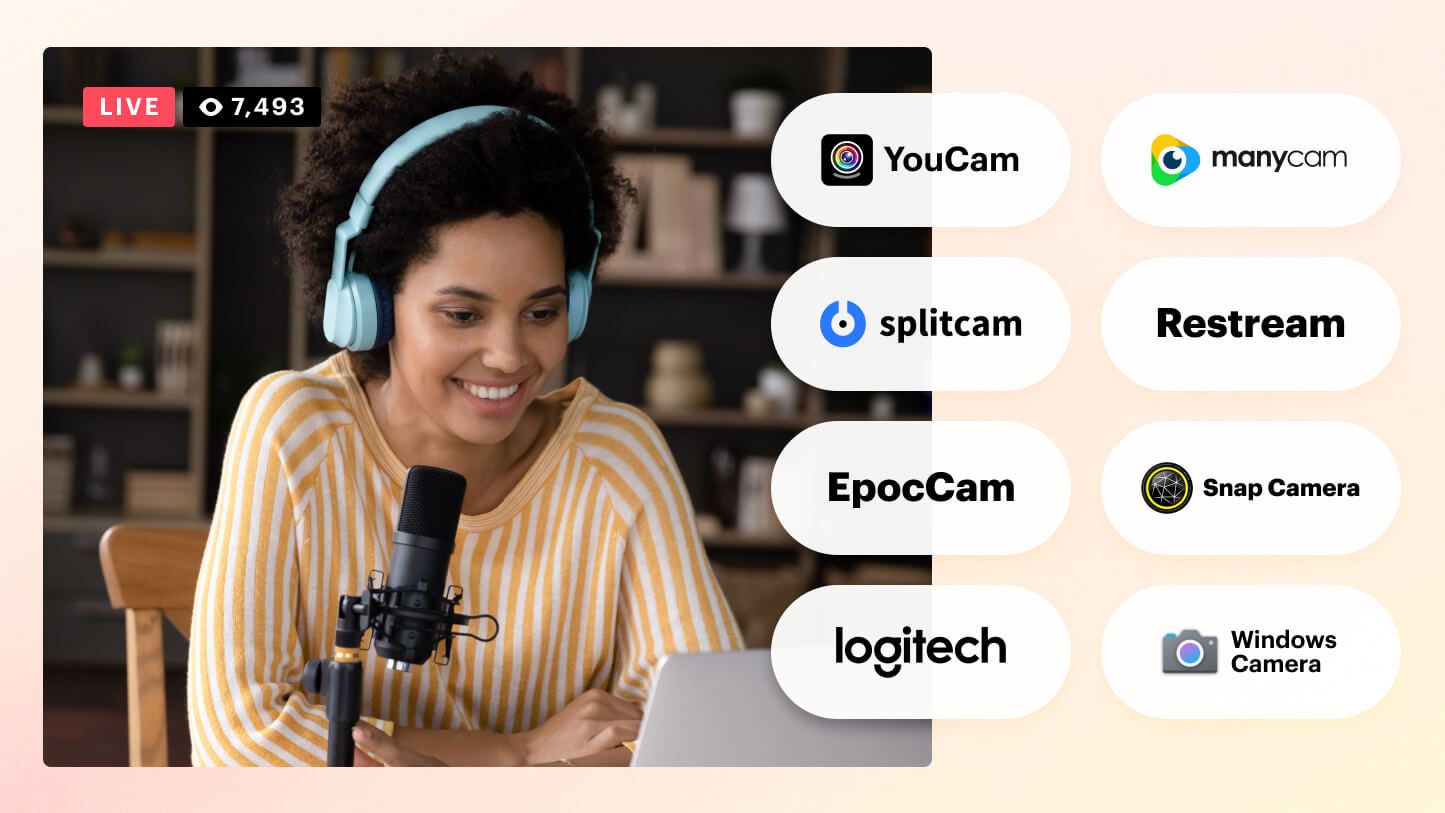This detailed image shows a young black woman with short, tightly coiled black hair, wearing light blue headphones and a yellow-and-white striped shirt. She is smiling and looking down at a silver laptop on a desk, speaking into a thick black desk-mounted microphone. She is seated in a wooden chair, with dark, blurry wooden shelving in the background and a cream-colored backdrop. In the top left corner, there is a red bar with white text that reads "LIVE," and beside it, a black rectangle displaying the number "7,493" indicating her viewers. On the right side of the image, partially overlaying her photograph, are two vertical columns of white oval icons representing different camera applications: Ucam, Splitcam, Epochcam, Logitech, Manycam, Restream, Snap Camera, and Windows Camera. These icons appear clickable, suggesting links to the respective camera services or products. The setting suggests a live-streaming session, possibly an online advertisement or webcast interface.